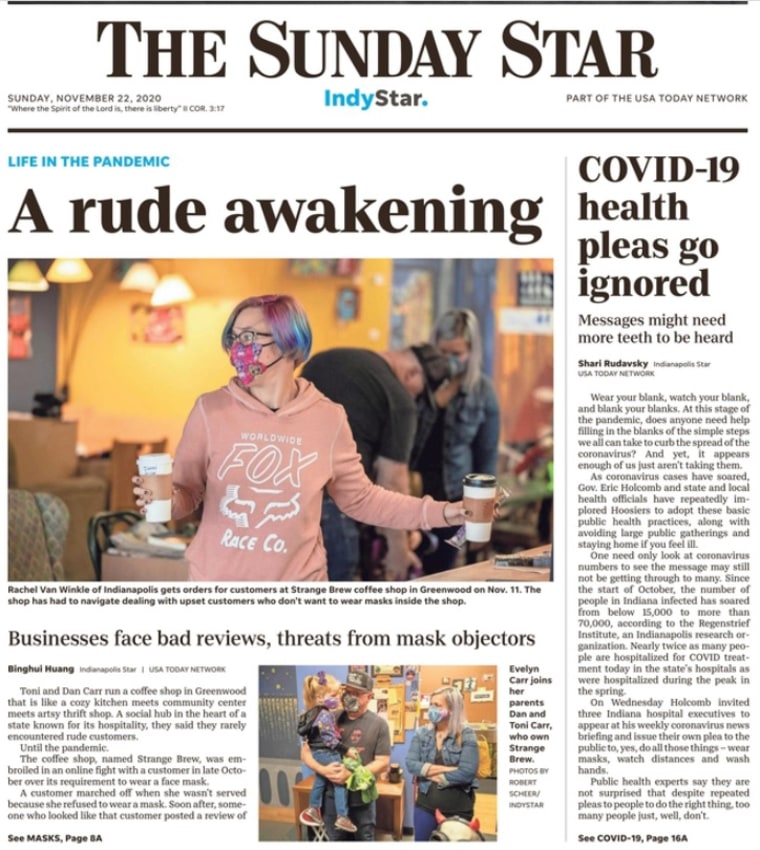This cropped screenshot captures the front page of the Sunday Star from November 22, 2020. Dominating the layout at the top is the title "Sunday Star" in prominent black font, accompanied immediately below by "Indy Star" aligned to the right, both a part of the USA Today Network, indicated in smaller black text. The date "Sunday, November 22, 2020" is inscribed at the top left.

A thick black line demarcates the header from the body of the newspaper. In the top-left section of the page, the headline "Life in the Pandemic" stands out in bold blue font. Below this, the subheading "A Rude Awakening" is printed in large black letters. Central to the layout is a sizeable image featuring a woman wearing a face mask in a coffee shop, accompanied by a brief caption in small black font beneath the photo. 

At the bottom of this segment, the bold black text announces "Businesses Face Bad Reviews, Threats from Mask Objectors," followed by the article text. Also featured is another thumbnail image towards the center-bottom of the page, depicting a family all wearing face masks.

To the right, a vertical panel contains another news article highlighted with the headline "COVID-19 Health Please Go Ignored" in bold black font, capturing another critical aspect of the ongoing pandemic.